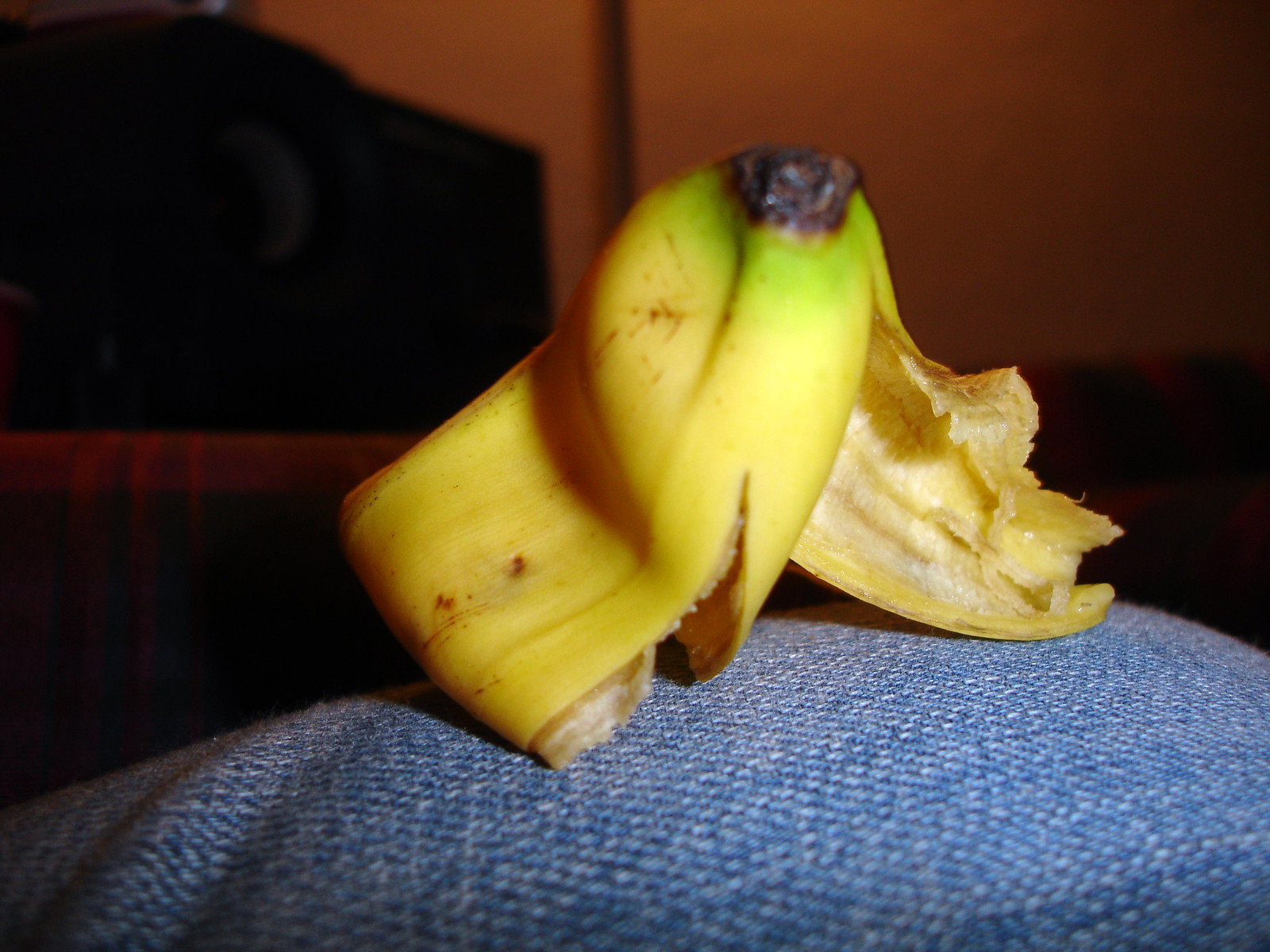This image offers a detailed, close-up view of a discarded banana peel. The background is predominantly dark, making it challenging to discern the exact color of the wall, which appears orangish due to the interplay of shadows. On the left side of the image, a brown object is visible, resembling the headboard of a bed, though its exact identity remains uncertain.

Dominating the scene, the banana peel rests atop what appears to be a pair of jeans, likely suggesting someone's leg or simply a jean-clad surface. The peel displays a brownish tip with a surrounding green ring, transitioning into yellow. It exhibits signs of aging with brown spots and subtle lines, clearly split open to expose the mushy, unappetizing interior, indicating the banana has been entirely consumed. The image's composition is accentuated by a pronounced shadow on the right side, adding depth to the overall composition.